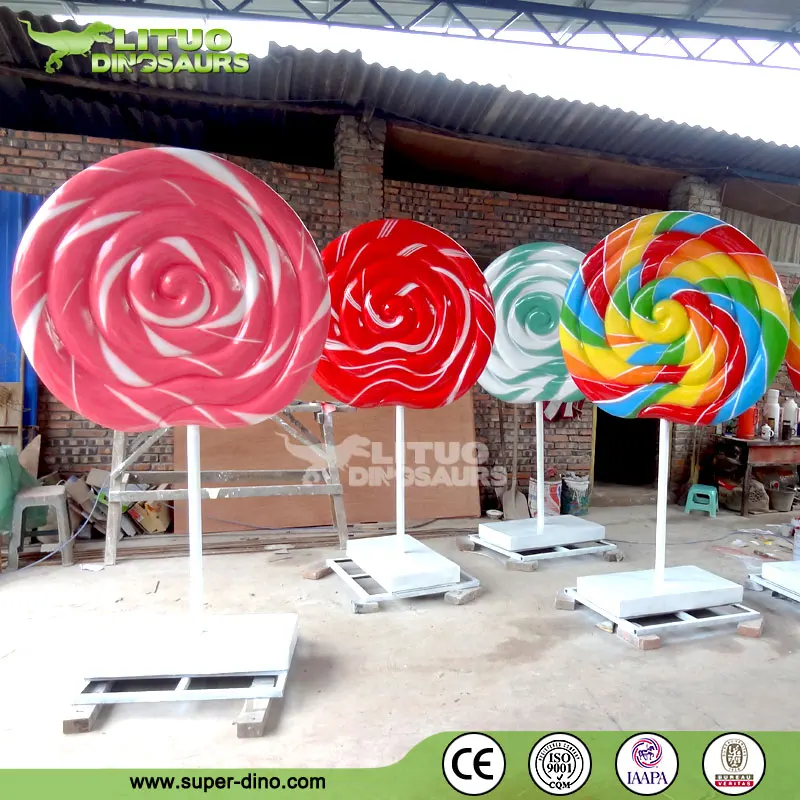This vertical rectangular photograph features a whimsical display of giant lollipops in front of a building. The lollipops, clearly artistic depictions and not real sweets, are mounted on white sticks and stand on white platforms or skids. Each lollipop boasts a vibrant swirl design, with one pink and white, one red and white, one mostly white with teal, and a rainbow-colored one featuring red, orange, yellow, green, and blue. The large size of these lollipops makes them appear larger than life, likely taller than an average person. In the background, a green dinosaur image accompanied by the text "L-I-T-U-D" is visible in the upper left corner, possibly hinting at a dinosaur-themed attraction or museum. At the bottom of the image, a green border displays the website www.superdino.com, suggesting a thematic link to dinosaurs. An open doorway and a small stool are seen behind the rainbow lollipop, adding to the scene's playful and fantastical setting.